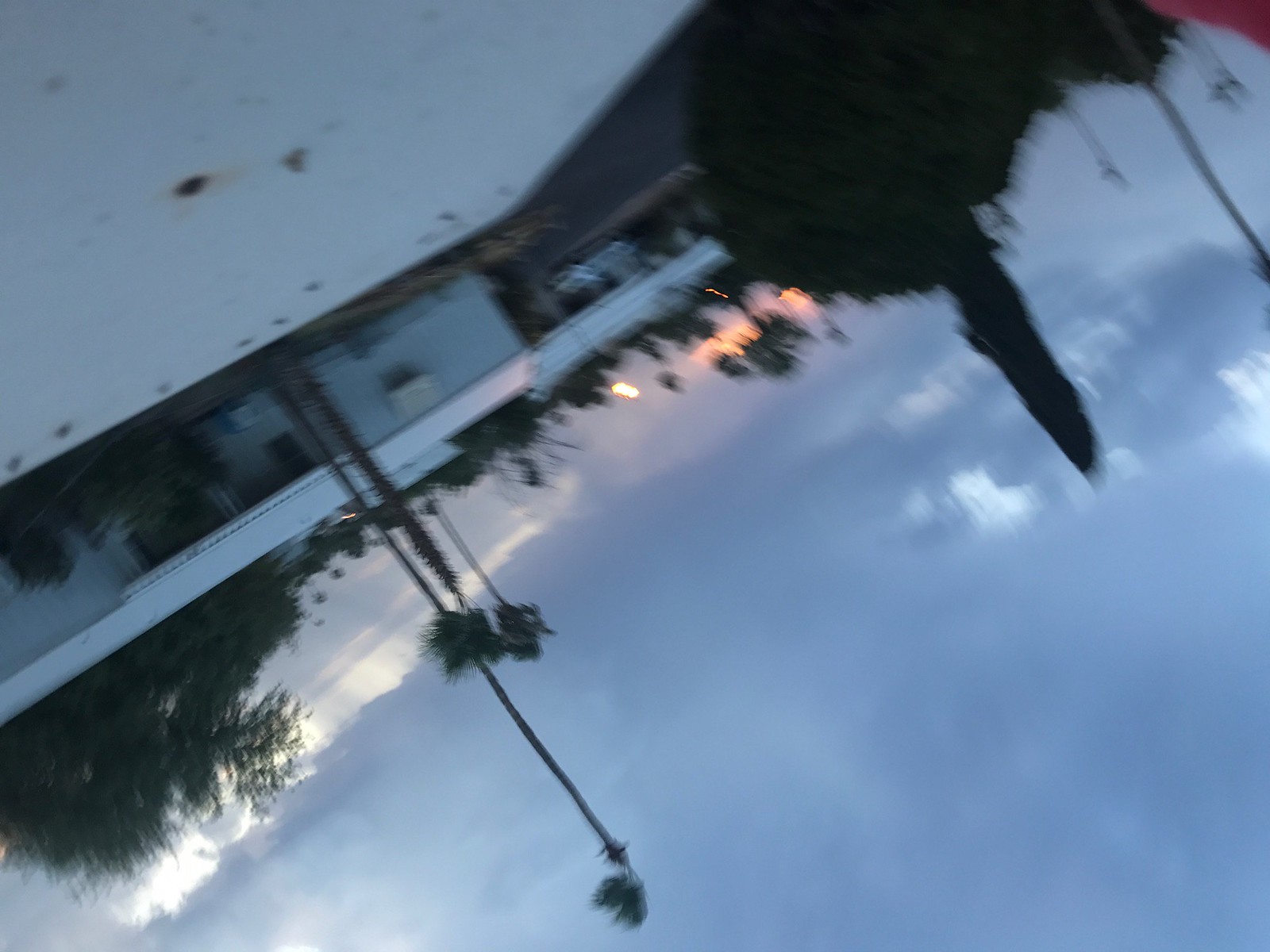The color photograph, initially upside down and now right-side up and slightly tilted, depicts a mobile home park with white trailers lined along broad streets. In the foreground, three tall, thin palm trees sway vigorously in the wind. The background showcases additional low white trailers, their roofs nearly blending into the cloudy sky above. The overcast sky, heavy with gray clouds, appears to be raining in the distance, with streaks of water visible against the blurred scenery. An orange tint colors a portion of the clouds, suggesting a setting or rising sun. Blacktop driveway areas weave between the trailers, and a solitary white car is parked in front of one of the trailers. The photograph seems to be captured from the vantage point of a white, flat rooftop, adding to the slightly sideways orientation of the image. Hints of poplar trees and blurry buildings can be seen off to the side, contributing to the overall impression of a serene yet windblown mobile home community.